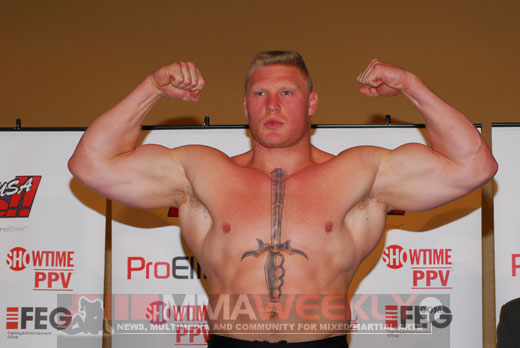The image depicts a highly muscular and ripped professional athlete posing confidently at an athletic event. Positioned center stage, he stands with arms raised, flexing his massive biceps and chest, exuding a very serious demeanor. The athlete, who is suggestively a Mixed Martial Artist based on the "MMA Weekly" text visible on a transparent banner at the bottom of the image, is shirtless, revealing a large greyish sword tattoo that stretches from below his neck to just above his navel. His flat top blonde haircut, blue eyes, and ruddy red complexion add to his striking appearance. The background features white banners adorned with text and logos, including "Showtime PPV FEG Pro," against a backdrop of beige, pink, red, black, white, gray, tan, and blonde colors. His attire is completed by black pants, although only visible above the waist. The image captures an intense, focused moment, showcasing the athlete's formidable physique and presence.